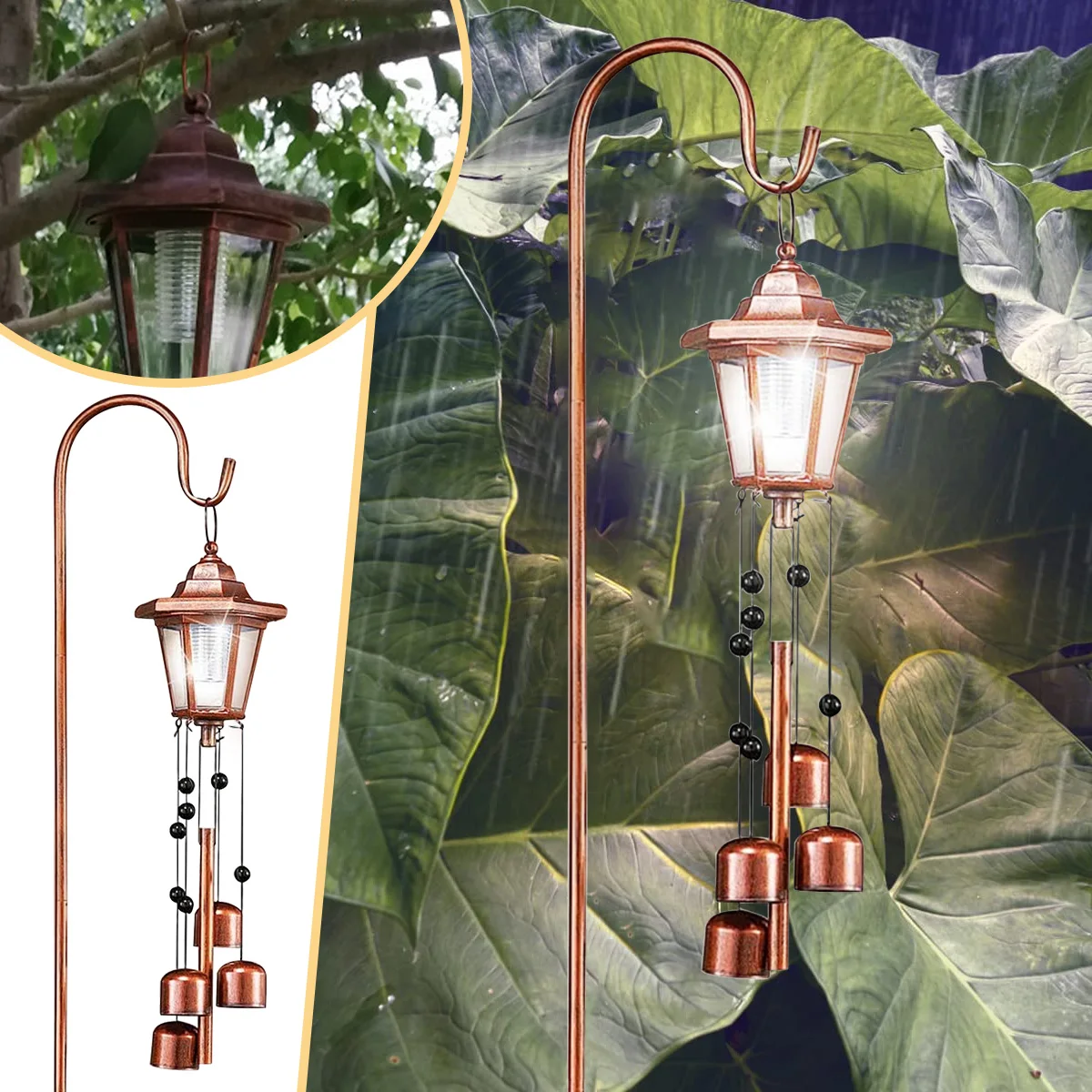The image is a detailed advertisement showcasing elegant garden or path lights that double as wind chimes. The focal point is a sophisticated copper lantern with 4 or 5 clear glass panels surrounded by copper borders, suspended from a gold, shepherd's staff-style hook. Decorative beads and bells hang beneath, adding charm and functionality. The lantern, part of a wind chime ensemble, includes metal wires and brass cups that strike a central brass cylinder when moved by the wind. This entire arrangement is staged against a backdrop of lush, large leaves, likely either elephant or banana leaves, adding to the serene, natural setting. In the primary outdoor scene, the lantern is beautifully illuminated, possibly under rainy conditions given the visible smudges or smears around the light, enhancing its glow. The advertisement also includes a close-up of the wind chime's top section and a separate view of the wind chime against a plain white background for added clarity.